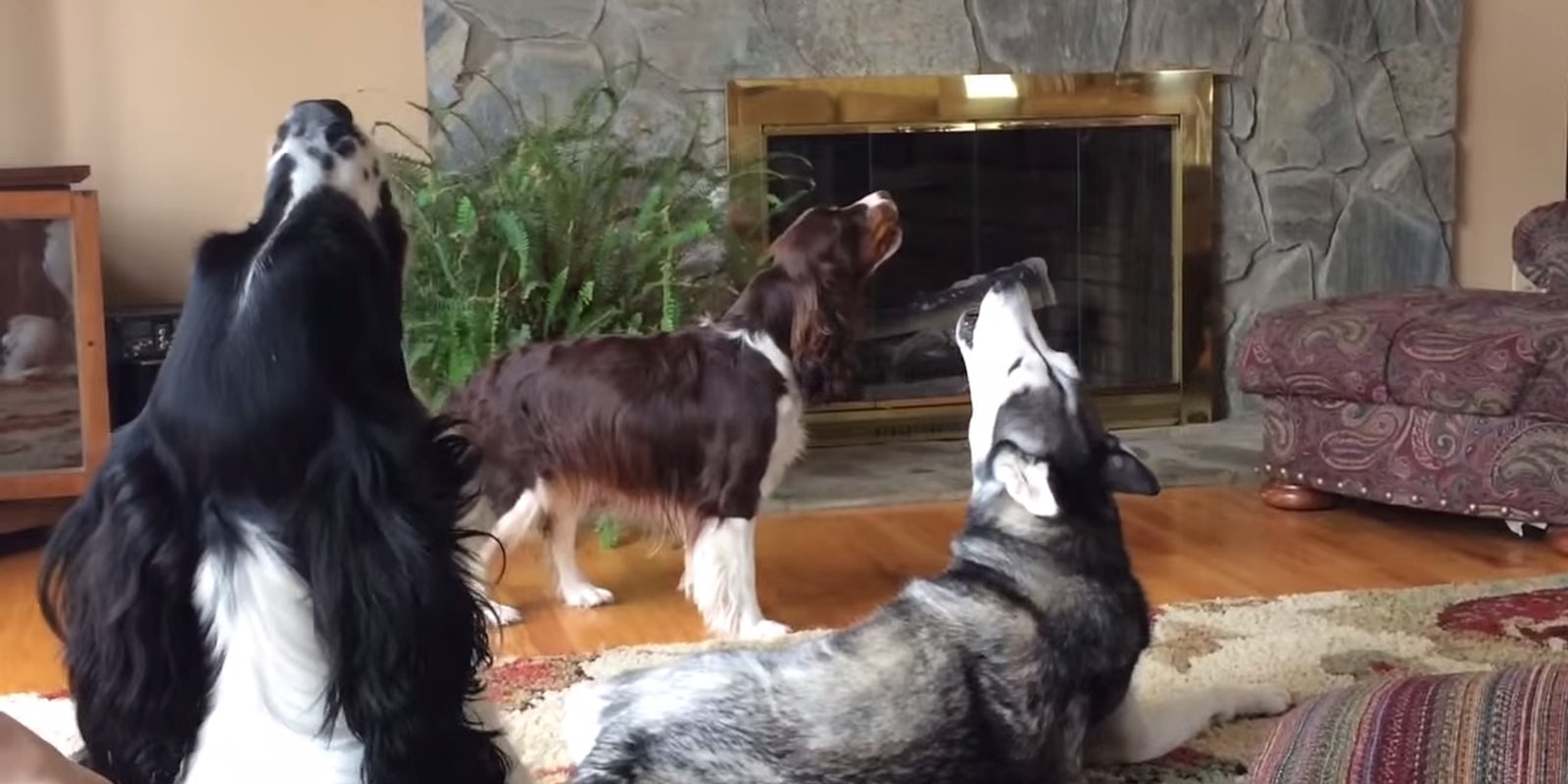In the image, you see a cozy and detailed living room setting. The focal point is a trio of dogs, each caught in the act of howling with their heads thrown back and mouths open towards the ceiling. The first dog appears to be a Husky with black, gray, and white fur, lying down while howling. The other two dogs resemble Collies or Spaniels, with one being brown and white, lying on a carpet, and the other black and white, standing nearby. All three dogs showcase distinctive breed characteristics and contribute to the lively scene.

The room features a prominent fireplace adorned with cobblestones and trimmed in gold, exuding a warm, rustic charm. Next to the fireplace, a green plant adds a touch of nature. To the side, there is a wooden floor and a side table. A paisley-patterned purplish burgundy chair or couch, which has a blanket draped over it, sits near the fireplace, complementing the overall cozy atmosphere. The dogs are positioned on a tan carpet woven with subtle greens and reds, enhancing the room's warmth and homeliness.